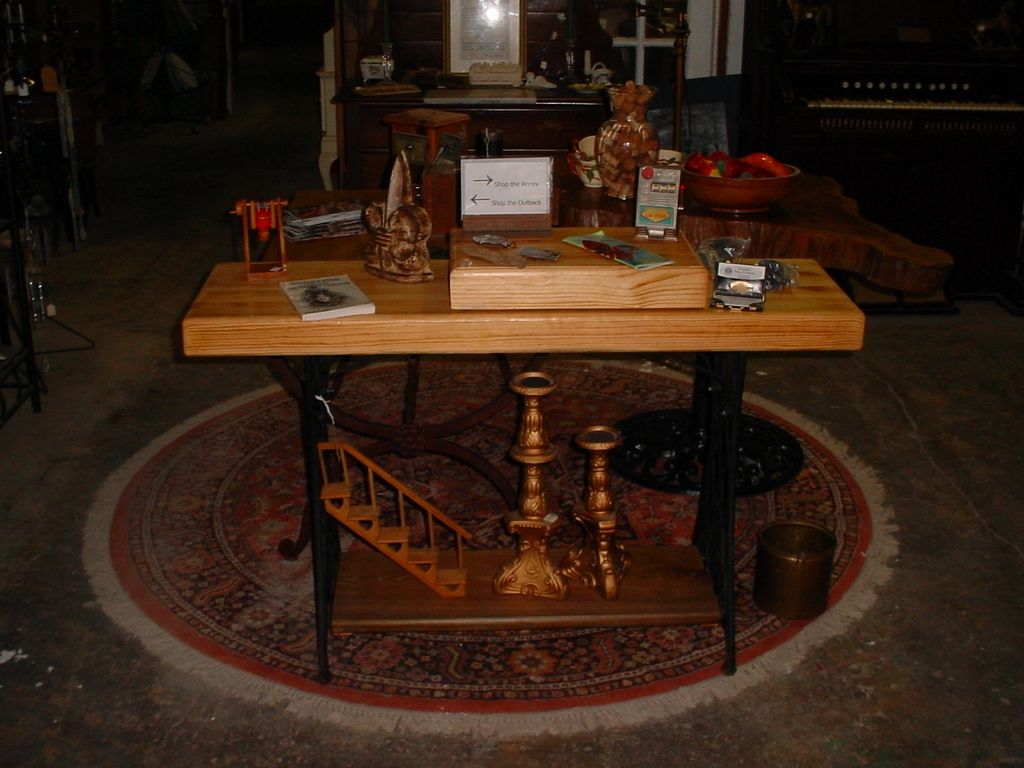The image depicts a highly detailed and eclectic setting within what appears to be an antique store or a collected space in a home. Dominating the scene is a medium-sized wooden table with a light brown rectangular top, supported by wrought iron legs and a lower shelf. On this lower shelf, there are two mismatched candlesticks—one taller than the other—likely made of brass or copper, along with a small decorative wooden staircase.

The tabletop is cluttered with various antique items, including a book and an assortment of peculiar objects. Among these are a small red figurine and a mysterious brown object resembling two pretzels with a spike. A wooden square is also present, holding additional unidentified items. Beside the table, a cylindrical dark brown container reminiscent of an old coffee can adds to the vintage atmosphere.

Beneath the table and surrounding areas lies an ornate, Persian-style rug featuring intricate patterns with red, tan, and dark brown or black hues. Behind this primary table stands another piece of furniture resembling a natural wood slice table, also supported by wrought iron elements. This table holds a brown vase and a wooden bowl filled with multicolored items in red, yellow, green, and purple.

In the background, there appears to be a piano organ and a visible cross, possibly part of a window's design. This setting is filled with various artifacts and objects, embodying the essence of a space rich with history and collectibles.